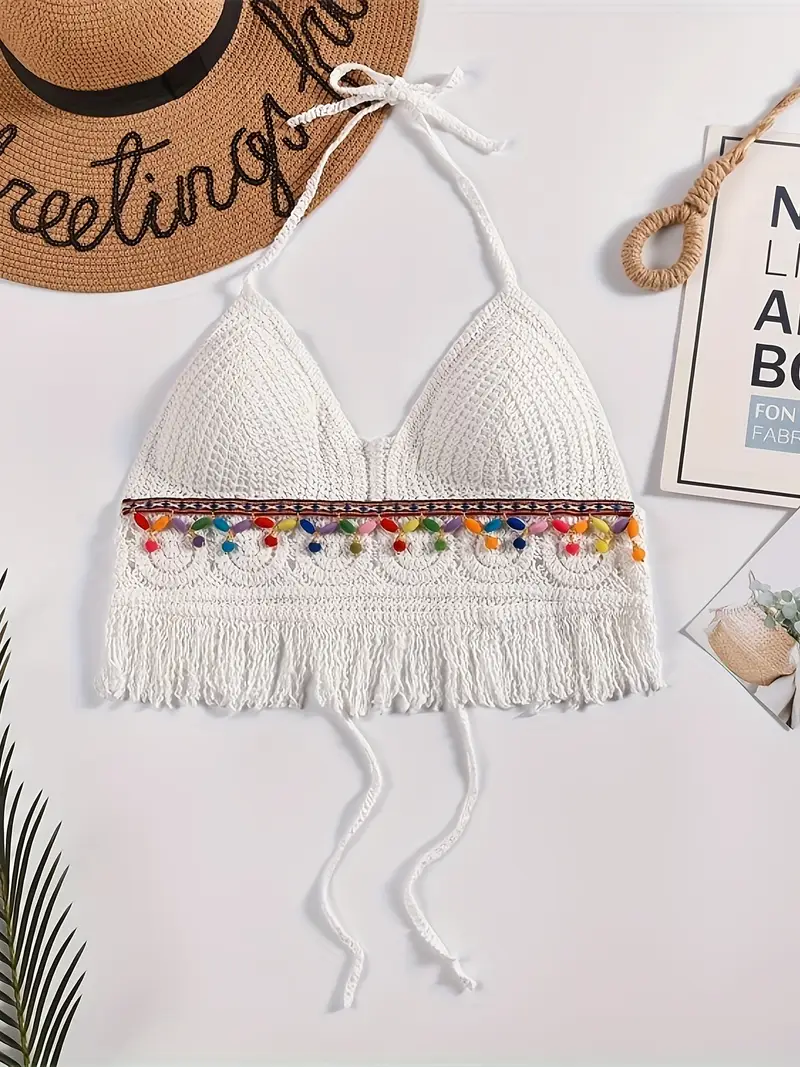The image is a vertically aligned photograph that prominently features a knitted white tankini top hanging on a plain white wall. The top has a bikini-style cut with spaghetti straps that tie behind the neck, and additional ties hanging down that would secure it around the back, leaving the back exposed. Decorating the piece, just below the bra cups, is a horizontal strip of colorful beads in red, orange, green, blue, yellow, and gray. Below this patterned strip, fringe-like threads dangle from the bottom edge of the top.

Also hanging on the wall in the upper left corner is a straw hat with a wide brim, only partially visible. The hat features a black ribbon around it and partially visible text starting with "Greetings from...". In the top right quadrant of the image, there are glimpses of some cards or small signs with text and images, as well as a beige rope. A large palm leaf, presumably from a potted plant, slightly peeks into the frame from the lower left corner, adding a touch of greenery to the otherwise minimalist setting.